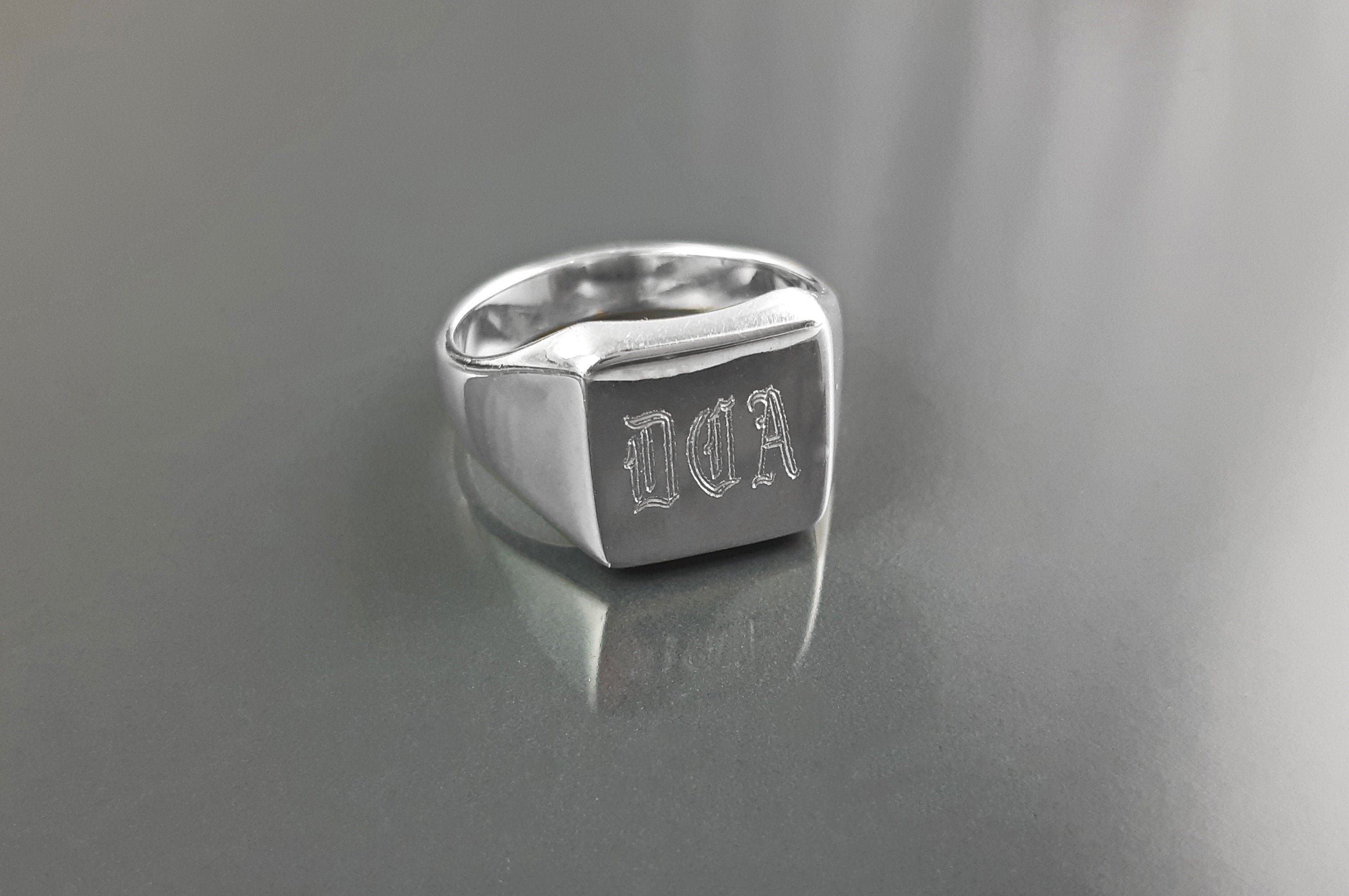This black-and-white photograph depicts a shiny, silver-colored ring, likely made of stainless steel, positioned centrally on a reflective, metallic flat surface. The ring, possibly a men's ring, features a prominent, flat top surface adorned with intricately designed letters "DCA" or "DOA" in a medieval or old-style font, which appear smooth and polished, enhancing their reflectivity. The band of the ring, though partially visible, recedes in focus due to the emphasis on the ring's detailed front. The reflective quality of both the ring and the metallic surface below creates a mirrored image, contributing to the photograph's striking visual contrast. There are no other elements present in the image, highlighting the ring as the sole subject.